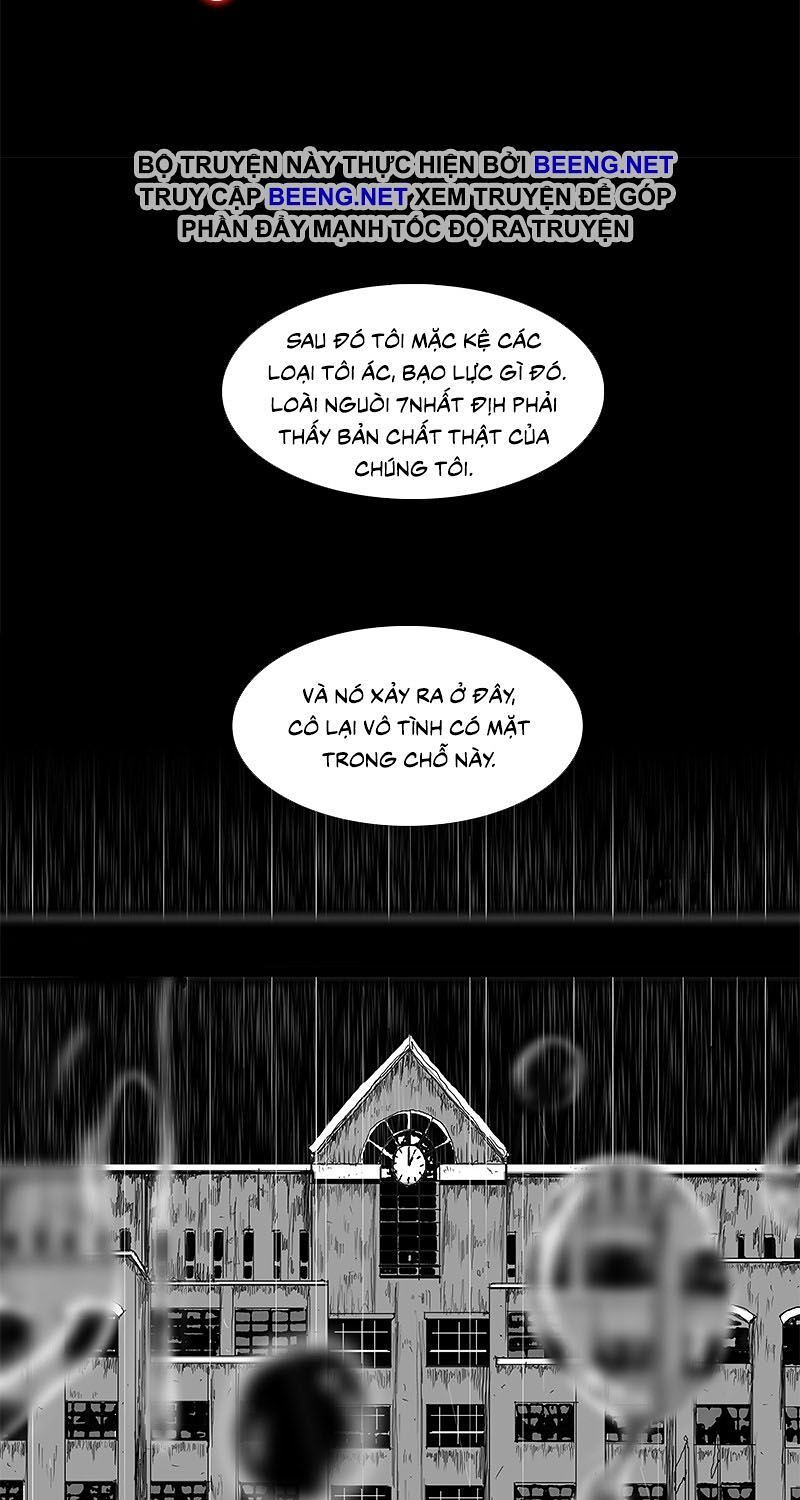The image resembles a page from a comic book or manga, featuring a vertically elongated rectangular shape. The top half is black with Vietnamese text outlined in gray, including the words "beeng.net" written twice. Below the black area, two white speech bubbles filled with black Vietnamese text are present. The bottom portion of the image depicts a detailed illustration of an old, rundown school building, characterized by a prominent roof peak with an arch window and a clock displaying one o'clock. The school illustration is rendered in black and white, spanning at least five floors with evenly spaced windows. The scene is overlaid with stylized raindrops or water streaks on glass, giving the appearance of rain falling or water running down a window.